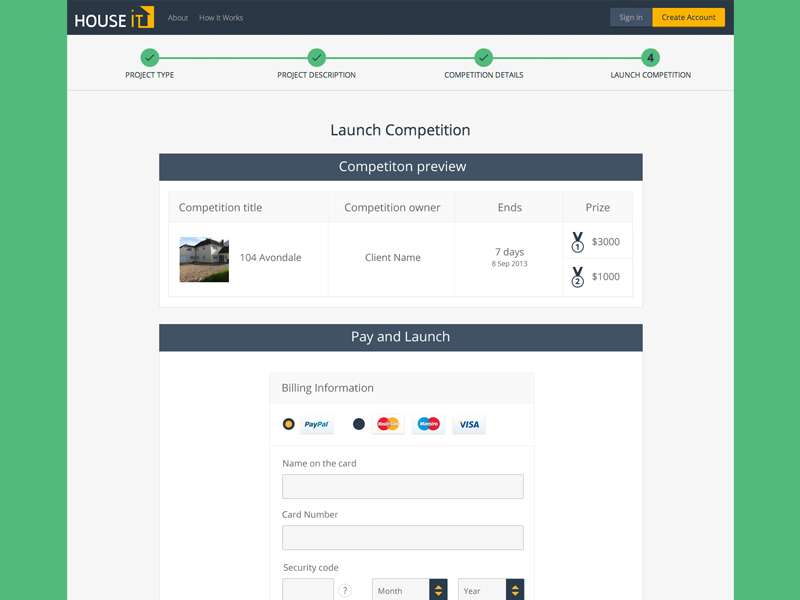The image depicts the homepage of a website called "Houseit." The website's logo features a white house icon with an orange "T" integrated into the design, creating the silhouette of a house. To the right of the logo, there are navigation tabs labeled "About" and "How It Works." Further to the right, users will find a "Sign In" button in gray and a "Create Account" button in orange.

Below the navigation bar, there is a progress section with several checkmarks indicating completed steps. The user is on the final step, "Launch Competition - Step 4," while the previous steps—Project Type, Project Description, and Competition Details—are marked in green.

Centrally positioned on the page is a headline reading "Launch Competition," followed by a "Competition Preview" section in white lettering on a navy blue bar. Below this, there are columns labeled "Competition Title," "Competition Owner," "Ends," and "Prize."

The competition title area features an image of a two-story white house with a grassy front lawn. The address "104 Avondale" is listed, along with the competition owner's name, the competition's end date of September 8, 2013 (ending in 7 days), and the prizes: $3,000 for first place and $1,000 for second place. Medals with "1" and "2" graphics indicate the respective prizes.

At the bottom, there are options to "Pay and Launch" the competition, accepting billing information from PayPal, MasterCard, and Visa. Users are prompted to enter their name, card number, and security code.

The main page has a white background, while the house icon bar features a dark navy blue background. Additionally, there are vertical green bars on each side of the page.